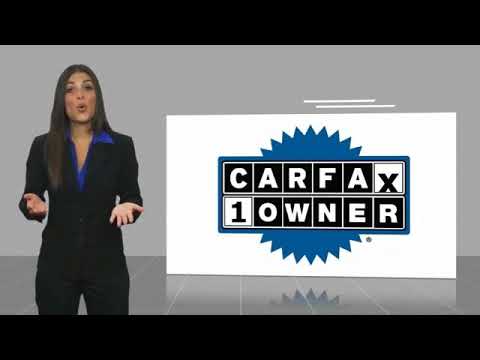The image appears to be a screenshot from an advertisement. On the left side stands a young woman with straight, long dark brown hair, wearing a black suit with large lapels and a blue blouse underneath. Her lips are slightly parted, forming an O shape, as though she is mid-speech. Her hands are partially outstretched with her palms up and elbows bent, gesturing as if explaining something. The background behind her is a uniform light gray color. 

To her right, there is a prominently displayed, large rectangular sign with a white background. The text on the sign reads "Carfax One Owner" in stylized black, checkered letters resembling the movable types on an odometer or an old-fashioned alarm clock. The 'X' in 'Carfax' appears as if it is ticking over. The sign is set against a blue sunburst pattern which adds a shiny effect with visible reflections. The edges of the image feature an inch-thick black band at both the top and bottom, framing the scene. Overall, the colors in the image are muted, including shades of blue, white, gray, black, and the natural skin tone of the woman. The entire image is somewhat out of focus and dark, suggesting it might be captured from a low-quality video or TV ad.